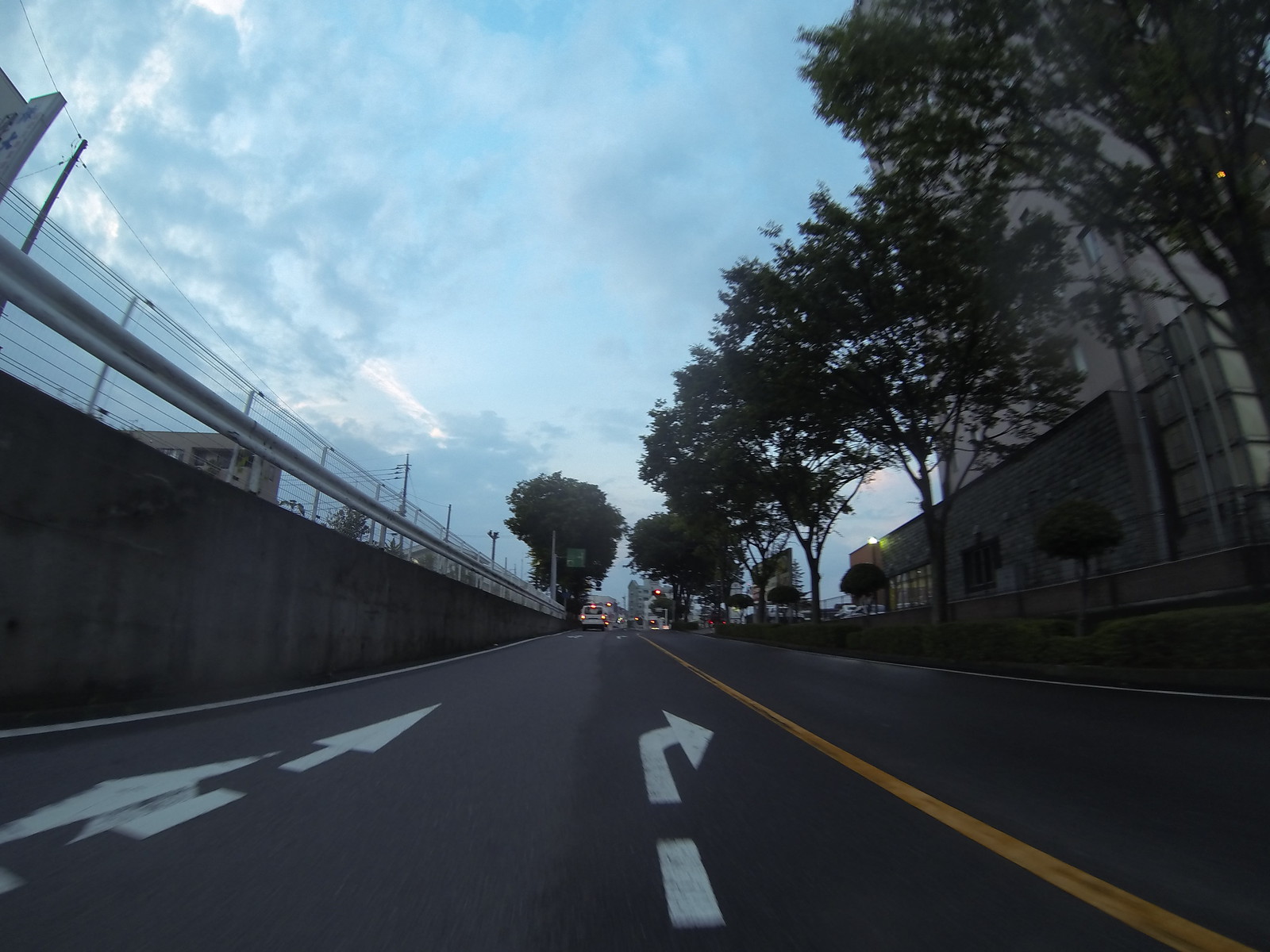In the image, the sky above is a vivid blue adorned with scattered clouds. Below, a broad expanse of asphalt stretches out on the ground, marked with directional arrows pointing left, straight ahead, and right, all highlighted in yellow. To the left, a sturdy concrete wall runs alongside the road, complemented by a metal railing. On the far right, a tall building with numerous windows stands majestically, partially obscured behind some trees. A row of cars proceeds forward, guided by stoplights, casting the scene in a somewhat somber, shadowy tone. The overall ambiance of the image is distinctly dark and moody, accentuated by the interplay of light and shadow.